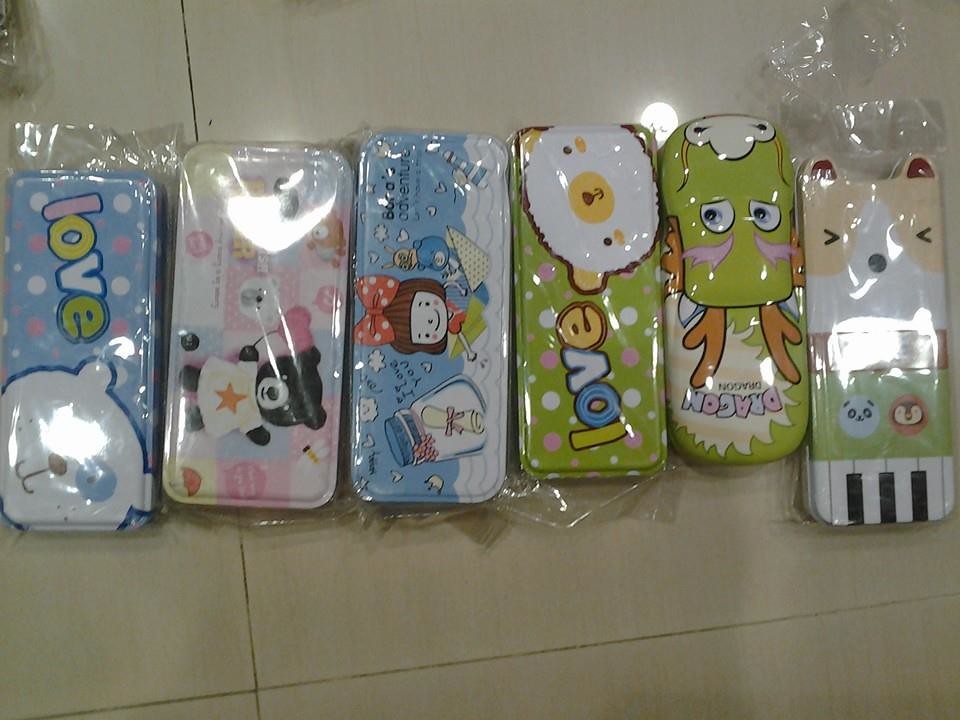The color photograph captures a close-up of six rectangular objects, which appear to be smartphone covers or pencil cases, arranged in a horizontal line on a tiled floor of beige to greyish-green hue. Each cover is wrapped in clear plastic except for the second one from the right, which is unwrapped. 

From left to right:
1. The first cover features a cartoon cat head with the word "love" written in multicolored letters. The background is blue with white and pink polka dots.
2. The second cover shows a black bear wearing a white t-shirt with an orange star, set against a pink background with circular designs.
3. The middle cover depicts a cartoon girl with a large red bow in her hair, shown with white dots. She appears to be in a boat on white water, with a jar containing a paper scroll next to her, all set against a blue background.
4. The fourth cover has "love" written in multicolored letters, accompanied by a green bear head with a yellow nose amidst green and white polka dots.
5. The fifth cover displays a green creature with brown legs and possibly horns, with the word "dragon" written near the bottom that’s hard to read.
6. The last cover features the head of what resembles a dog, beige around its eyes with white detailing and two ears at the top. There’s a green section at the bottom with tiny illustrations of a panda and a bird, and below that, piano keys in black and white. 

There is noticeable glare from a light source reflecting off the glossy plastic wrapping, enhancing the detailed textures and colors of the covers.